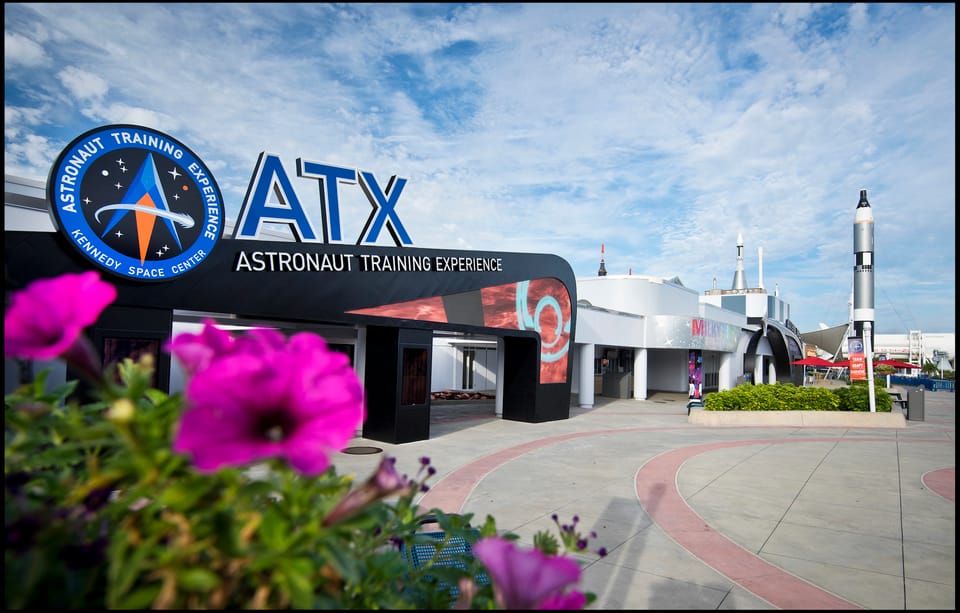This image captures the exterior of the Astronaut Training Experience (ATX) building at the Kennedy Space Center, Cape Canaveral. The ATX building is notable for its sleek black facade, adorned with large blue letters outlined in white that spell out "ATX." Adjacent to it is a substantial white structure, both of which are part of the Kennedy Space Center complex. In the background, multiple rockets are visible, standing tall as a testament to NASA's space endeavors. The outdoor setting includes a spacious concrete walkway, featuring red circular inlays that give the appearance of a bull's-eye from above. This pedestrian-friendly area is accentuated by vibrant purplish-pink flowers and greenery at the forefront, adding a touch of color to the industrial scene. The photograph, devoid of people, showcases the inviting public space designed for visitors eager to learn about space exploration and the astronaut experience.